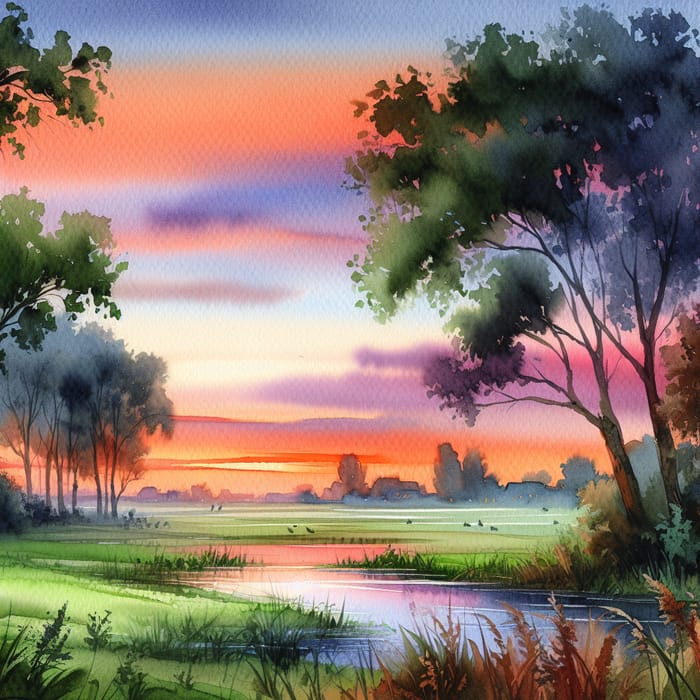The image is a hand-drawn watercolor painting capturing a serene, natural scene at sunset. In the foreground, there's a shallow, calm blue pond located towards the lower right-hand corner, bordered by large weeds and some brown ferns. The immediate surroundings of the pond are filled with thin prairie grasses, some orange and most green. The middle ground is dominated by an expansive, lush green meadow with birds depicted flying over it, and no trees in sight within this area. Flanking the meadow on both the right and left sides are tall, leafy oak trees typical of American deciduous forests.

In the background, a distant cityscape silhouette of houses and additional tree lines emerges, adding depth to the scene. Above it all, the sky paints a dramatic picture with its sunset colors—shades of orange, blue, purple, and bright yellow clouds vividly indicating the time of day. This radiant sunset coloration reflects beautifully on the surface of the pond, adding a cohesive and tranquil ambiance to the artwork.